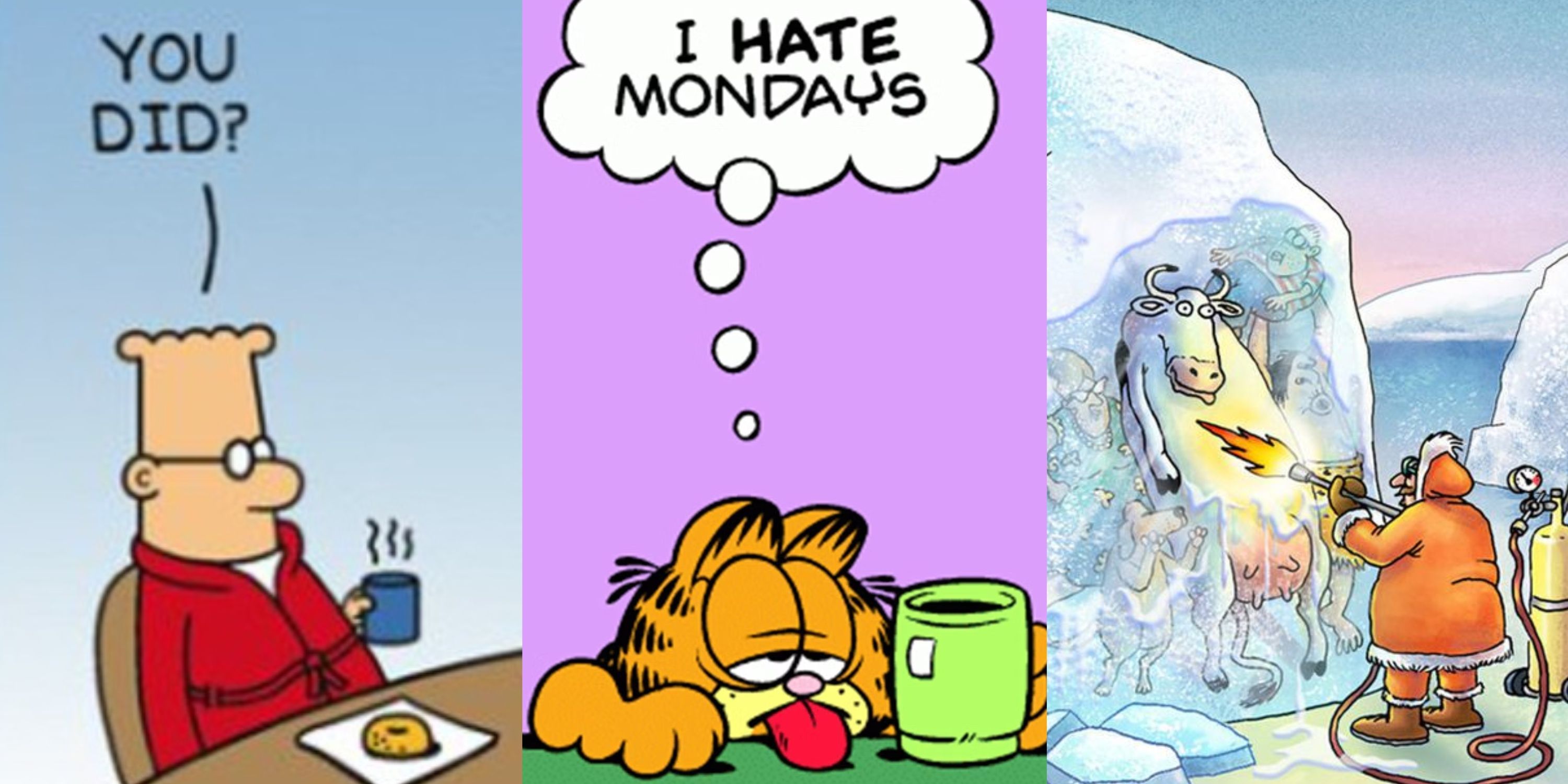This rectangular collage features three distinct comic panels. On the far left is a panel from Dilbert. In this scene, Dilbert is seated at a desk, donning a red robe with a white shirt underneath. He has a cylindrical head with some bumps indicating hair and wears thick, white-circled spectacles. In his left hand, he holds a blue coffee mug emitting steam, and there’s a donut on a napkin on the desk in front of him. A speech line above his head reads, "You did?"

The center panel showcases Garfield, the iconic orange tabby cat with black stripes on his ears. Garfield, with exaggerated cartoon features and mostly closed eyes indicating fatigue, leans against a green table while holding a green coffee cup with black coffee. His red tongue sticks out, underscoring his tiredness. Against a blue background, a thought bubble above him states in bold letters, "I hate Mondays."

The right panel depicts a scene reminiscent of The Far Side comics, set in a cold, arctic environment. A large, heavy-set man in an orange parka with white fur trim operates a flamethrower connected by a hose to a yellow gas tank with a pressure gauge. He uses the flamethrower to melt an iceberg that encases a cow, a dog, and what appears to be a woman and child, as well as a caveman. The cow and animals are frozen in an upright position, suggesting they were caught in motion. This final panel relies on visuals alone, without any accompanying text.